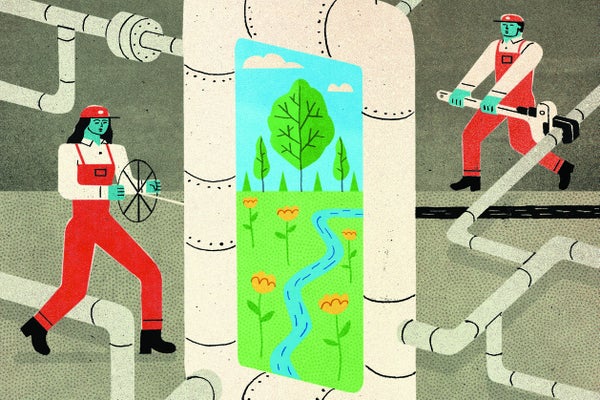This is a detailed, abstract, and cartoony-styled illustration depicting an industrial scene. At the heart of the image lies a complex, large rectangular structure composed of pipes with smaller pipes branching out to the left and right. The scene is set against a smooth grey wall on a pale beige-green floor. Centered on this large structure is a whimsical poster or portal featuring a vibrant natural landscape—a flowery meadow with red and yellow flowers, green trees with black trunks, a serene blue river winding through, and a bright blue sky with puffy white clouds.

Flanking this central industrial apparatus are two characters, each with blue skin, wearing white shirts underneath red coveralls, complete with red ball caps. The character positioned on the right side, distinguished by black hair, black boots, and a cap with a white dot and black brim, is seen holding a large, oversized cartoon wrench with a white handle and black hook, positioned on a grey pipe. This pipe extends downward in an S-shape and then in an L-shape towards the bottom right of the frame. On the left side, the other character, identical in appearance except for long black hair, is gripping a wheel that is attached to the left side of the rectangular structure. The entire background is filled with a maze of interconnected pipes, adding to the intricate industrial feel of the illustration.